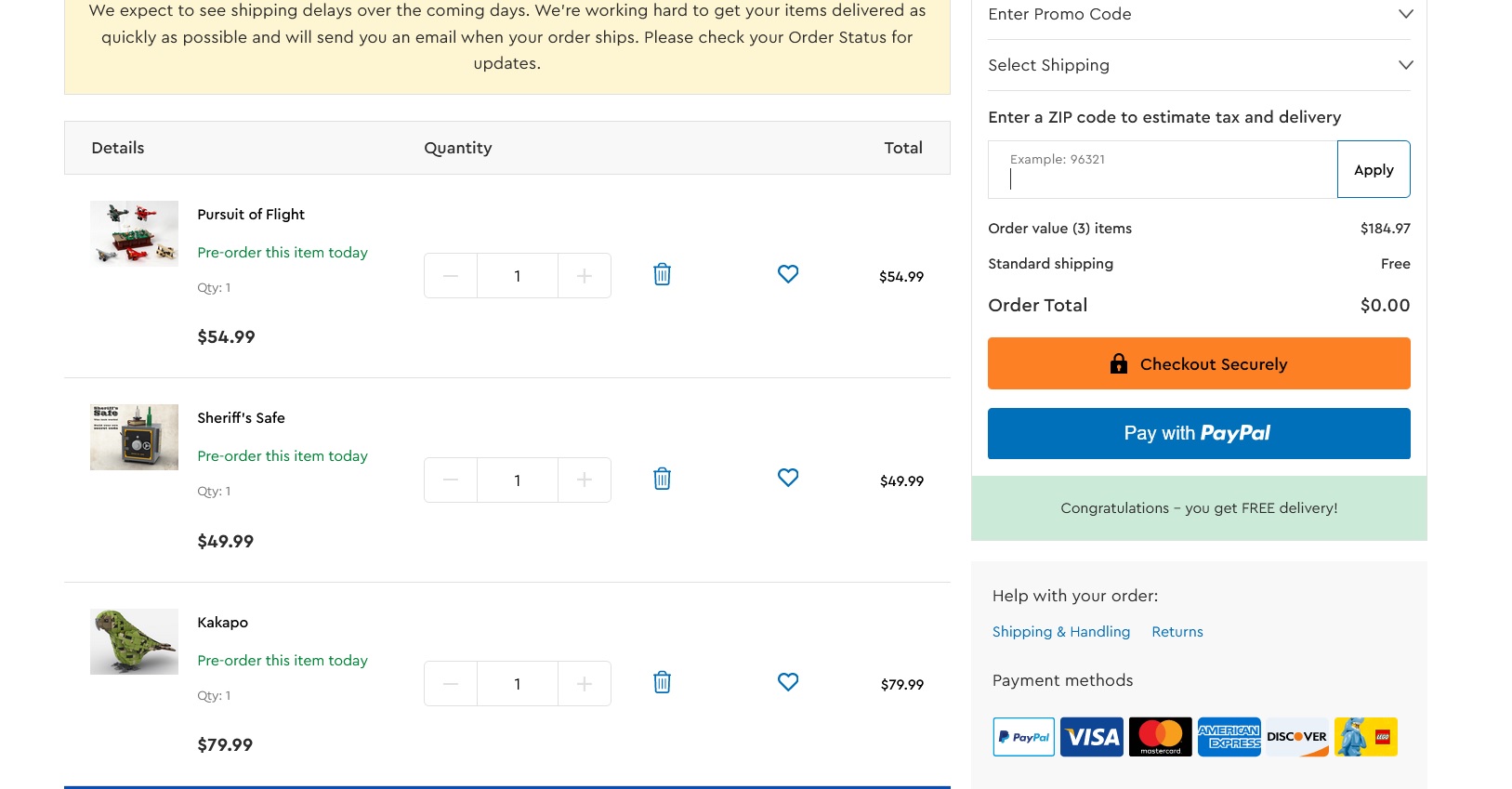The image displays a detailed shopping cart and checkout page on a website. At the top of the page, there is a status notice informing customers about potential shipping delays in the coming days. 

Occupying the left two-thirds of the image, the shopping cart section is organized into columns for product details, quantity, and total price. The first listed item is "Pursuit of Flight," available for pre-order at $54.99, with the quantity set to one. Users have the option to adjust the quantity, delete the item, or add it to a wishlist via a heart icon. The total price is displayed to the right.

Below this, another pre-order item, a "Sheriff's Safe," is listed at $49.99. Following this, there is an item named "Cuckapoo," depicted as a bird, priced at $79.99. It is unclear if this item is ceramic or not.

On the right side of the image, the order summary is presented. It includes sections for entering a promo code, selecting shipping options, and entering a zip code to estimate tax and delivery costs, along with buttons to apply these inputs. The order summary shows a value of three items totaling $184.97, with standard shipping marked as free, and the current order total displayed as zero.

Below this, there are multiple buttons including an orange "Check Out Securely" button and a blue "Check Out with PayPal" button. A blue banner congratulates the customer on their free delivery and provides links for help with the order, shipping, and handling information.

Payment options displayed at the bottom include PayPal, Visa, MasterCard, Amex, Discover, and another unidentified logo that might resemble Lego.